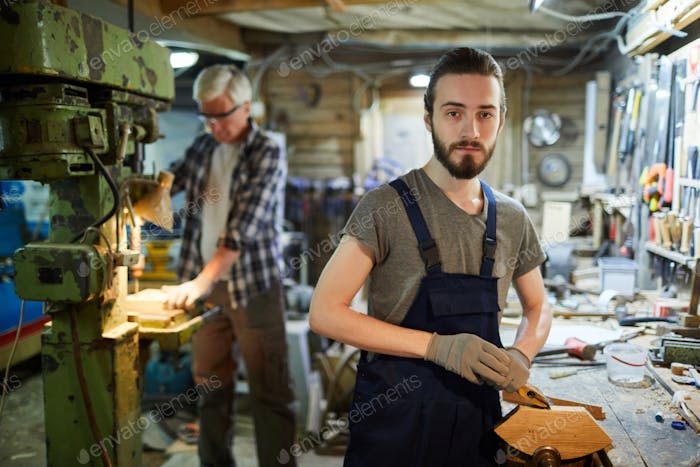The photograph captures a detailed scene inside a cluttered woodshop, featuring two men at work. Dominating the foreground is a younger man with short brown hair, a short beard, and a mustache with a goatee. He looks directly at the camera, his blue overalls layered over a gray t-shirt, his gloved hands busy sanding a wedged piece of wood on a messy workbench scattered with miscellaneous tools. Behind him, towards the left and slightly out of focus, stands an older man with white hair and safety goggles. Dressed in a plaid button-up shirt over a gray t-shirt and brown slacks, the older man operates a large, green, industrial drill press, its rusty exterior bearing chipped paint. The shop itself is packed with various tools and workbenches, contributing to the sense of industrious activity.